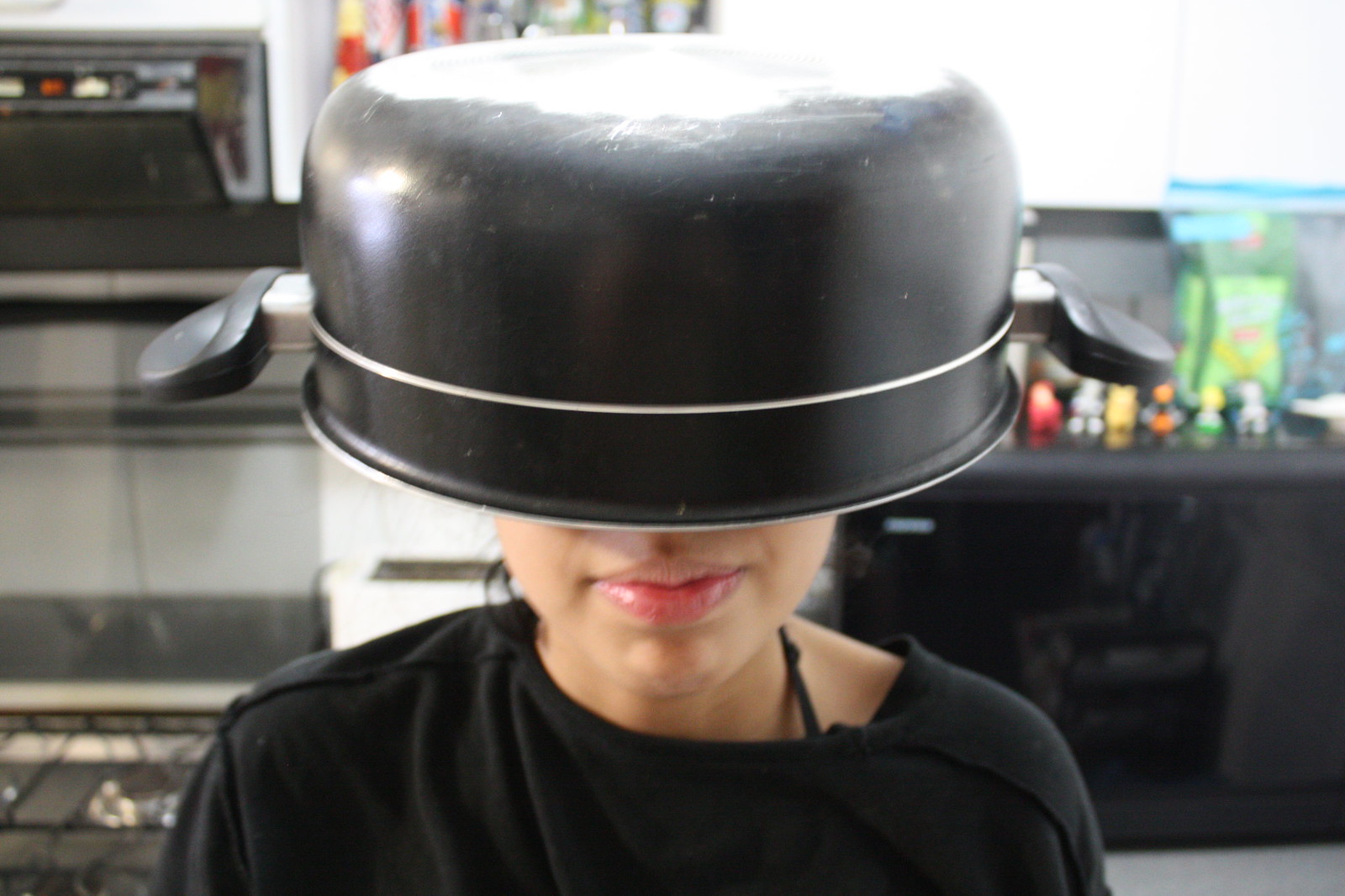This photograph depicts a young woman standing in a kitchen with a black cooking pot on her head. The pot, which has a silver stripe around its top edge and handles on either side, obscures her face down to just above her mouth, revealing only her nose, lips, and a few strands of her dark hair. She wears a black shirt, which seems to have a small string peeking over her left shoulder, and possibly pink lipstick on her full lips. The bottom of the photograph cuts off at her chest.

In the background, the kitchen environment is somewhat blurry but discernible. To the left of the woman, there's an oven and a tiled floor, with another white appliance nearby. Behind her head, obscured by the pot, a window with curtains can be seen, along with a counter beneath it cluttered with various items, including figurines like a Pikachu. To the right, there's another counter with a reflective black surface, possibly part of an appliance. Above this counter, shelves hold additional items, although these are too blurry to identify precisely. The scene is well-lit from above, casting a glare on the top of the pot and illuminating the area.